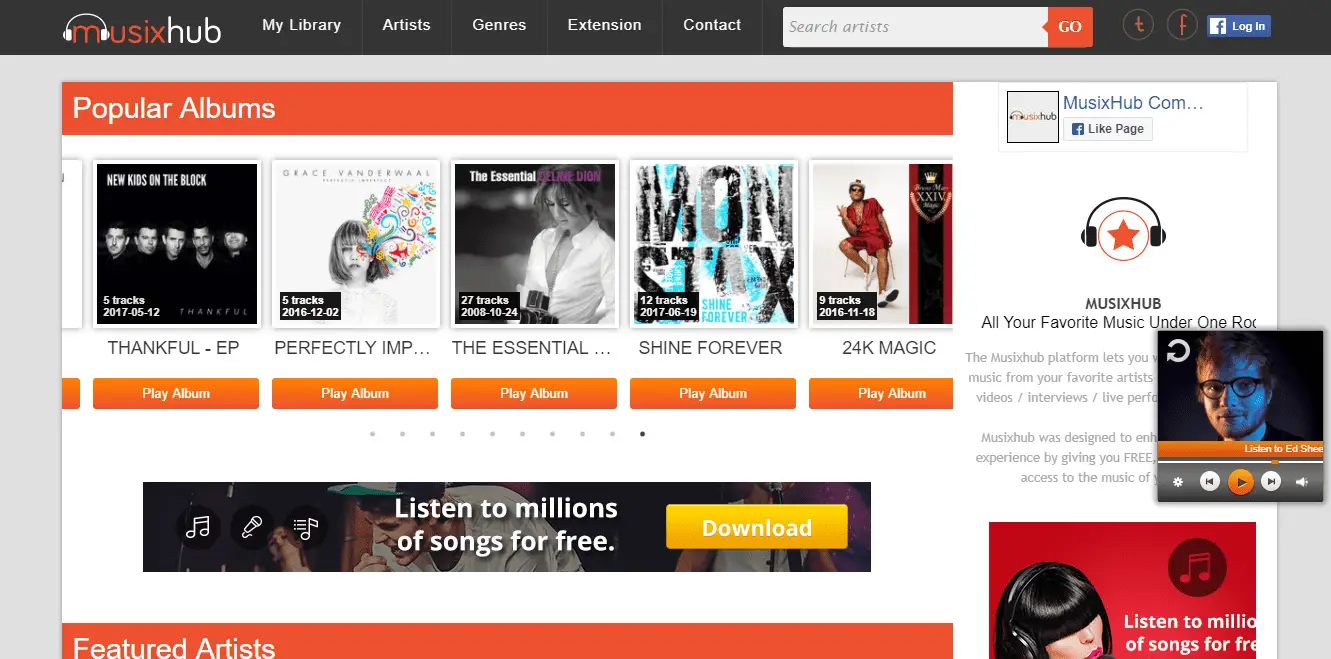In the image, the top left corner features a logo titled "MUSIX's Hub," with the letter 'M' adorned with a pair of headphones positioned above it. The word "MUSIX" is written in bold red letters, while "'s Hub" is in white. Adjacent to the logo on the right, a series of navigation tabs are displayed, including "My Library," "Artist," "Genres," "Extension," "Contacts," and a search bar accompanied by a red "Go" button. Below these, the "Enterprise" section showcases icons for Twitter, Facebook, and a "Facebook Login" option.

On the left side of the image, there is a section titled "Popular Albums" written in white text against an orange background. This section lists several popular albums. Each album is accompanied by an orange "Play Album" button below its title. The albums displayed include:
1. "Thankful EP"
2. "Perfectly Imperfect" - 5 tracks
3. "The Essential" - 27 tracks
4. "Shine Forever" - 12 tracks
5. "24K Magic" - 9 tracks

On the right side, a large text banner reads "Music's Hub: All your favorite music under one roof." Below this, a brief description appears, though it is partially obscured by the current playing music panel, which highlights "Listen to Ed Sheeran" and features play controls such as "Play Button," "Preview," "Forward," "Volume," and "Settings."

An advert is positioned below the music player, with a vibrant red background and a slogan that reads "Listen to millions of songs for free." It features a woman wearing black headphones, strikingly contrasted by her black hair. The text "Listen to millions of songs for free" is also present at the bottom left of the image adjacent to a prominent yellow "Download" button.

Lastly, the bottom left corner of the image includes a "Featured Artist" section, indicated by white text over an orange background.